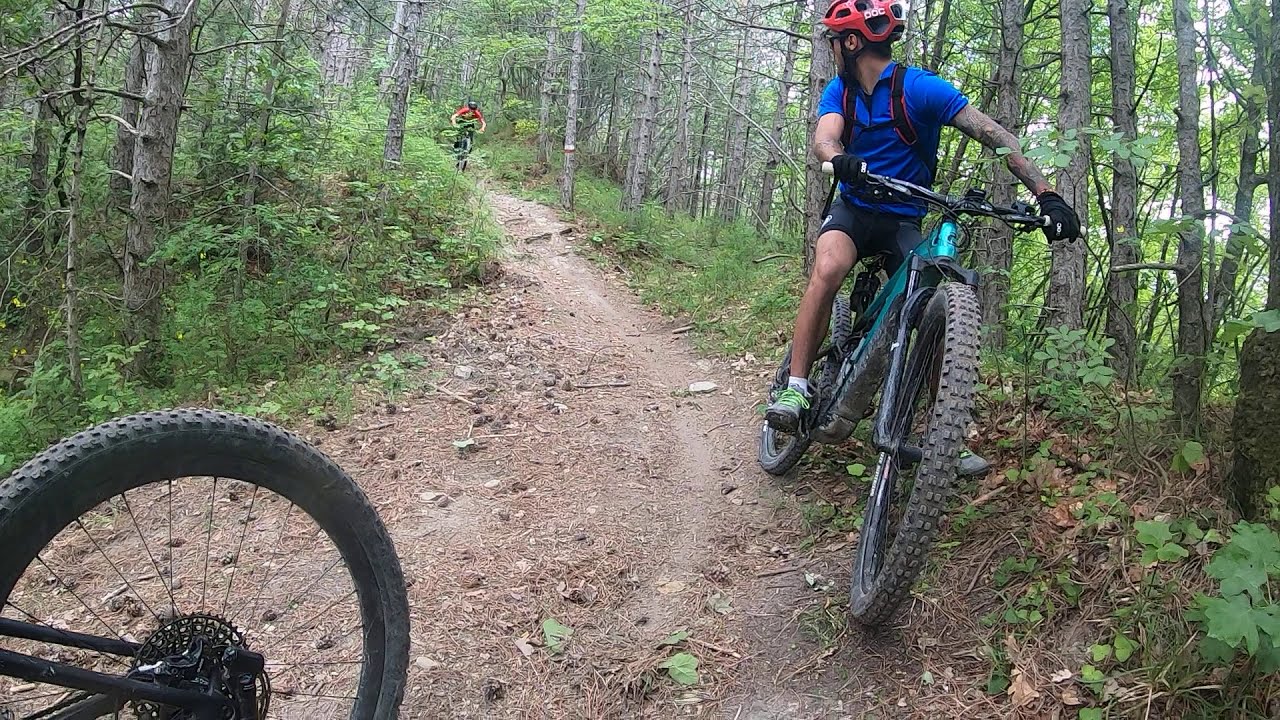In this detailed outdoor scene, we observe a group of three mountain bikers on a narrow forest trail, surrounded by pine trees. The trail, dotted with pine cones and rocks, runs directly through the center of the image. At the bottom left corner, we see the back tire of a bicycle. To the right, a gentleman on a teal-colored bike has paused, looking back over his shoulder down the path. He sports a blue collared shirt, fingerless black bike gloves revealing tattoos on his right arm, and green bicycle shoes. Farther back on the trail, another cyclist, clad in a red bicycle shirt and black helmet, is making his way down a steep incline. The scene, devoid of any text, features a palette of black, gray, green, blue, and red hues, capturing a vibrant moment in the woods during the day.